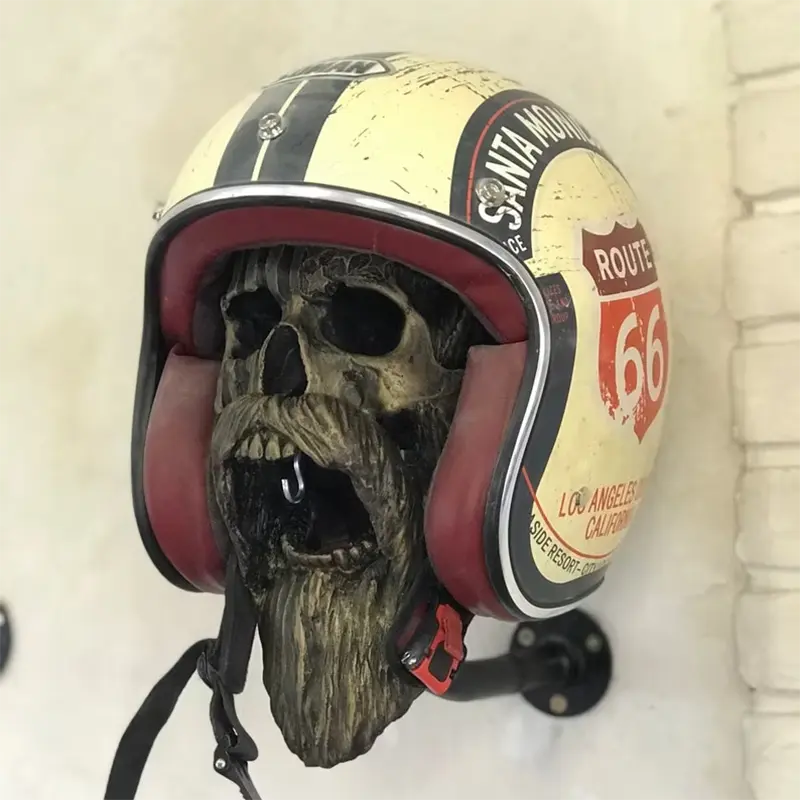The image showcases an aged and battered motorcycle helmet adorned with a vintage design, prominently featuring Route 66, Santa Monica, Los Angeles, California decals on its sides. The helmet, which has a yellow exterior with black racing stripes and maroon-red leather padding inside, encapsulates a bronze-colored skull, complete with a long beard and mustache. A silver hook is conspicuously placed inside the skull's open mouth. The helmet and skull ensemble is mounted on a black industrial pole, affixed to a whitewashed brick wall, adding to the eerie, almost surreal vibe of the photographic composition.